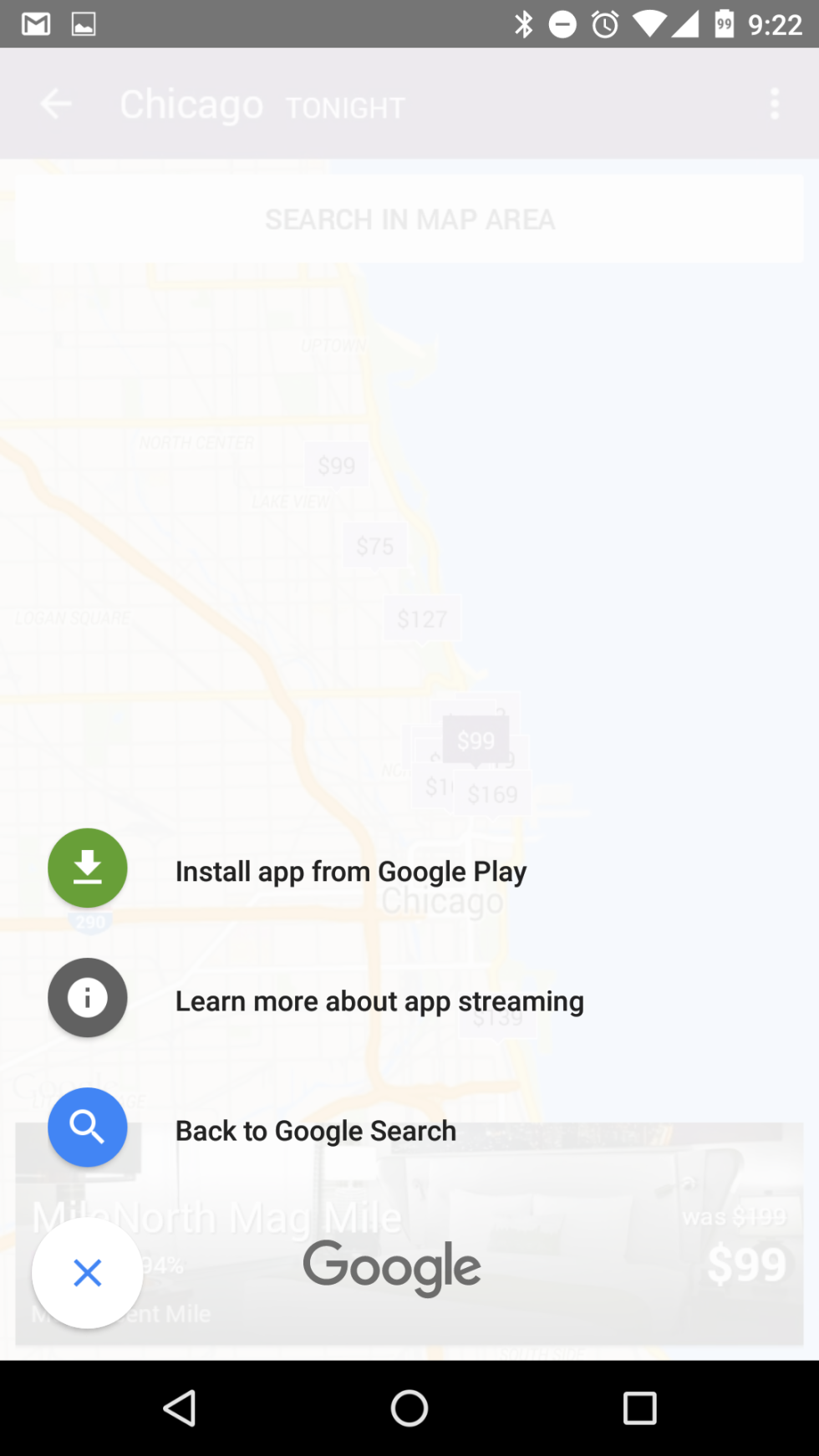This is a detailed caption of the screenshot taken from a phone:

The upper half-inch of the screenshot features a dark gray status bar. On the left corner, the Google Mail icon is visible, followed by the Google Photos icon. On the right side of the status bar in white text, the time reads 9:22. Also on the right, there's a battery icon showing 99% in black, full internet signal bars, full Wi-Fi signal, and an activated alarm clock icon. Additionally, a white circle with a black dash indicates an active Bluetooth connection.

The remaining area of the screen has a hazy overlay due to a pop-up tab. Through this haziness at the top, there is a left-pointing arrow with the text "Chicago Tonight" in white below it. Below this, there's a search bar labeled "Search a map area." The map itself is faintly visible but heavily obscured by the overlay.

Just past the midway point on the left side, a green circle with a download icon is present. To the right of this, the black text reads "Install app from Google Play." Below, there is a black circle containing a white "i" for information and to the right, black text reads "Learn more about app streaming."

Further below, a blue circle with a white search icon is present, followed by the black text "Back to Google search." Additionally, a white circle with a blue 'X' symbol appears ,with the black text next to it reading "Google."

At the very bottom of the screen, the navigation bar includes the back button on the left, the home button in the center, and the recent apps button (square) on the right side.